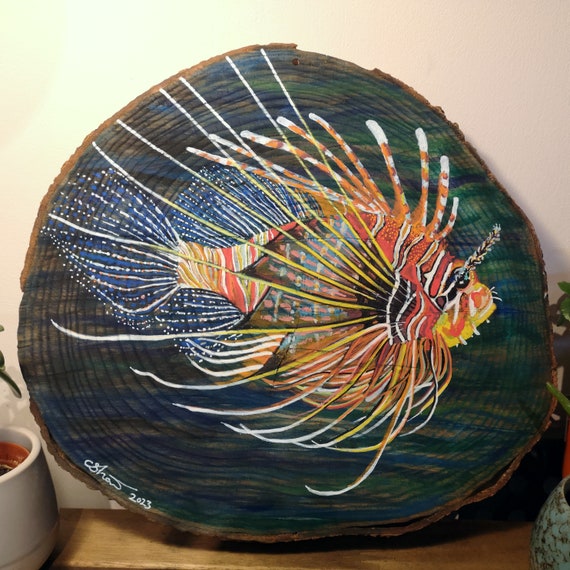This photograph captures a detailed artwork on a large, rustic tree trunk slice, showcasing its intricate wood grain and concentric tree rings. The slice is painted a vibrant blue and features a spectacularly colorful lionfish with its head facing right. The lionfish exhibits a striking combination of orange, white, blue, yellow, and pink hues. Its body is adorned with spiky tendrils and webbed fins, with orange and white striped spikes on the top, and a yellow bottom lip. The creature's mesmerizing fins and tail are blue with white stripes, and its face includes distinctive red, yellow, and white stripes highlighted by a black eye. In the lower left corner of the artwork, there is a white signature with the year, likely "2023". This stunning piece of art rests on a brown wooden table, flanked by a partially visible white planter on the left and a grayish-blue vase on the right, adding subtle context to its setting.